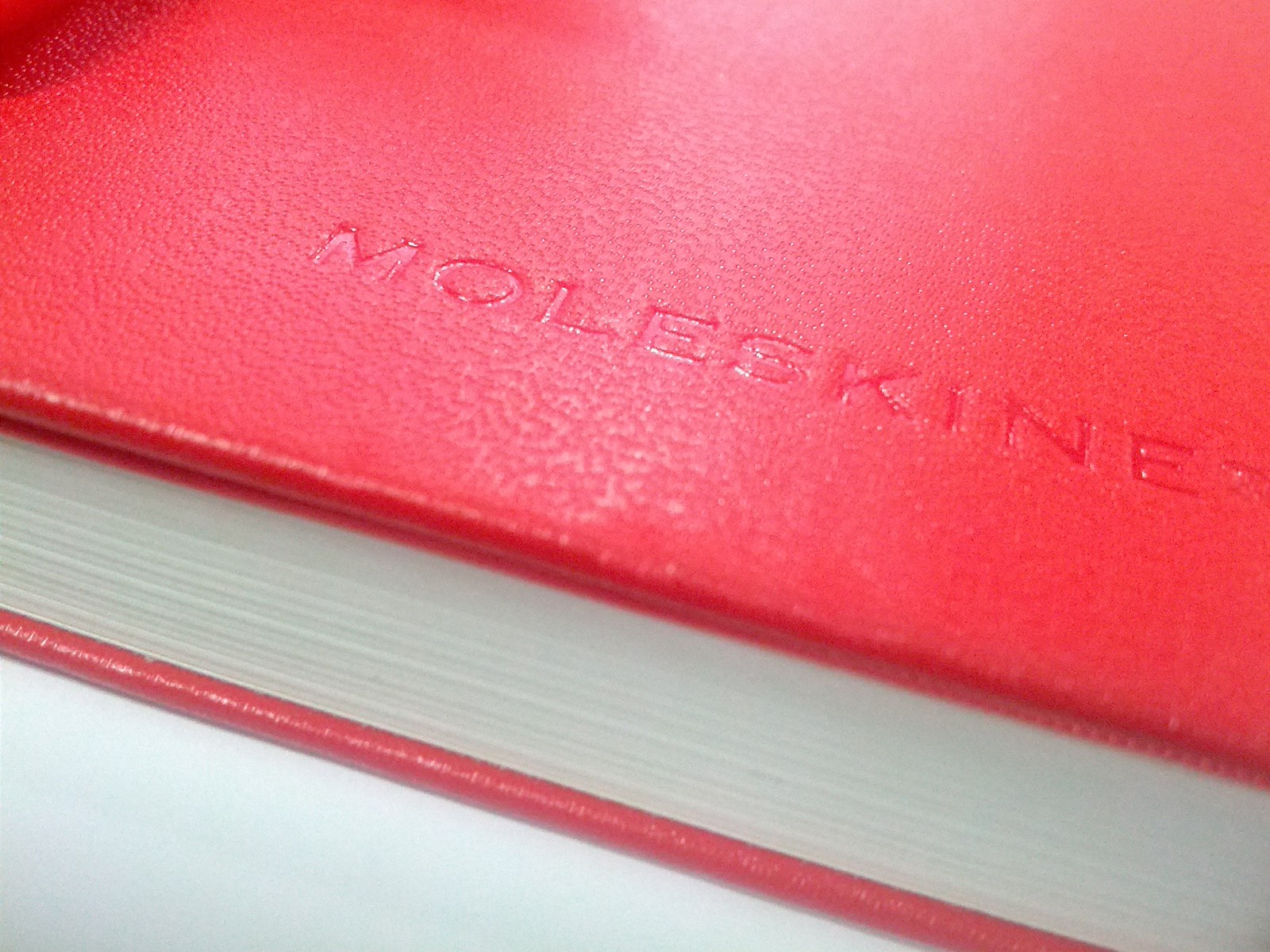The image showcases a vibrant, close-up view of the bottom section of a bright red Moleskine notebook. The notebook, which appears to be a journal, features a cherry-red, hardcover with a slightly textured, leather-like finish, making it somewhat rough to the touch. The meticulous lighting highlights the embossed "Moleskine" logo, especially illuminating the letters "mole." The visible section of the notebook reveals pristine, white pages, giving the impression of a thick stack, at least an inch or more, suggesting the notebook contains over 100 pages. The vibrant scarlet hue of the cover and the focused perspective on the bottom part of the journal emphasize its premium quality and detail-oriented design.